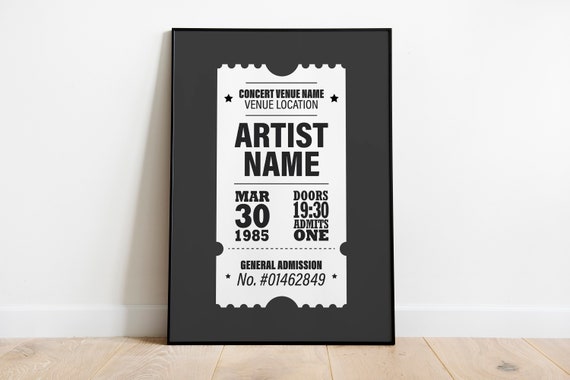This image captures a photograph of a concert ticket replica, framed and leaning against a white wall with a plain, light wooden floor underneath. The central focus of the photograph is a black-framed piece of black paper featuring a white ticket stub design. The ticket, which appears to serve as memorabilia, prominently displays details in bold, dark text. The information includes: the concert venue name and location, artist name, the date "March 30th, 1985," and the notation "Doors 19:30." It states "Admits One" on both ends and has "General Admission" followed by the ticket number "01462849" at the bottom. The classic ticket stub is designed with torn edges, adding to its authentic appearance.